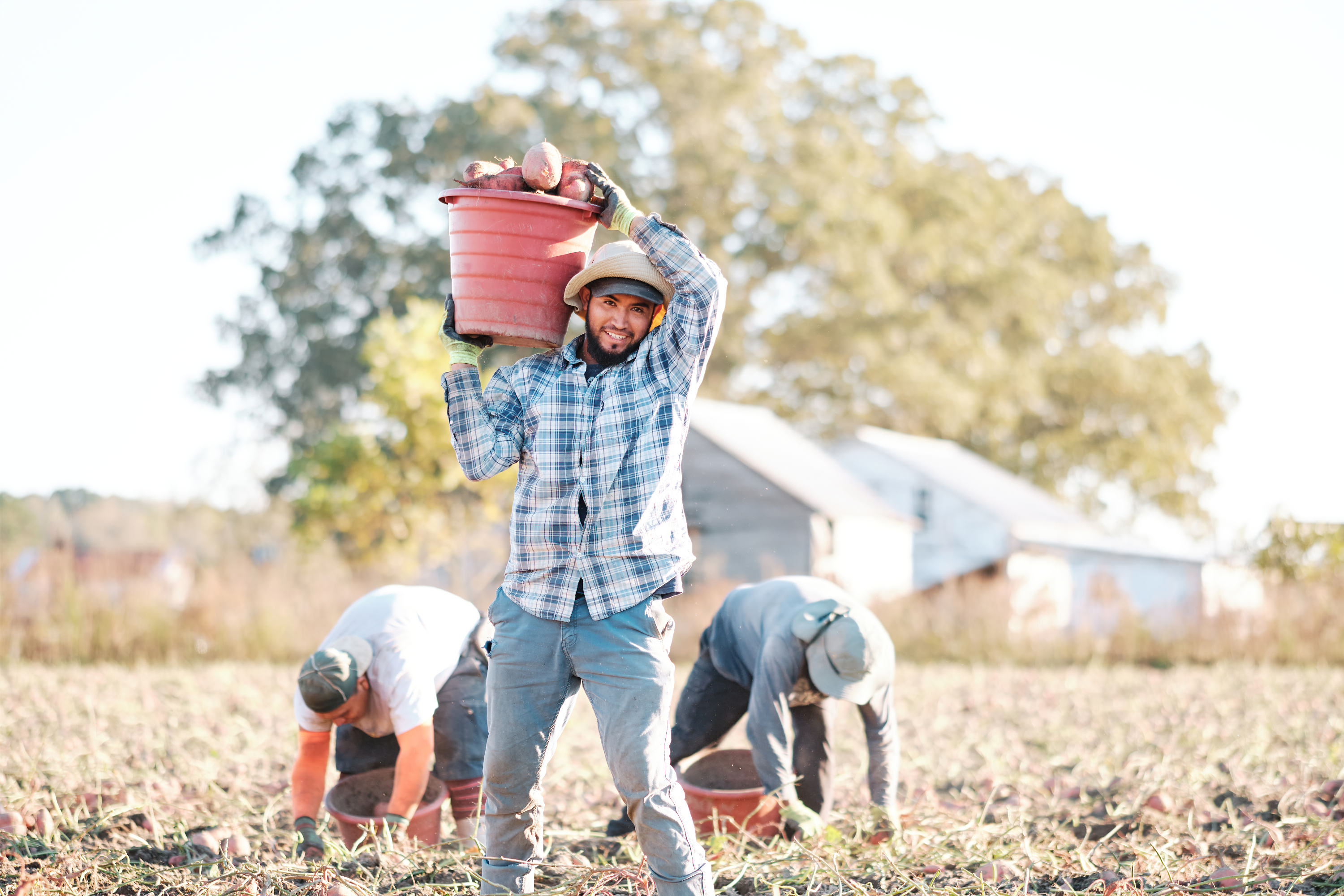In the image, three farmers are working diligently in a sunlit yam field. Centered in the picture stands a young man wearing a blue and white checkered long-sleeve shirt with a collar, beige pants, a white hat layered over a blue hat, and holding a pinkish bucket filled with large red yams above his right shoulder. His bearded face and focused expression convey the labor-intensive nature of their task. Flanking him are two workers, one to his left and the other to his right, both crouching and deeply engaged in harvesting yams from the ground. The worker on the left wears a white t-shirt with orange sleeves, grey shorts, and a cap, while the worker on the right is dressed in a full-sleeve blue t-shirt, blue jeans, and a hat. Both have similar buckets filled with freshly picked yams in front of them. In the blurred background, there's a light white sky, some large trees, and structures that appear to be triangular-roofed houses or small huts. The expansive field around them is golden with hay-like vegetation, encapsulating a serene yet industrious landscape.